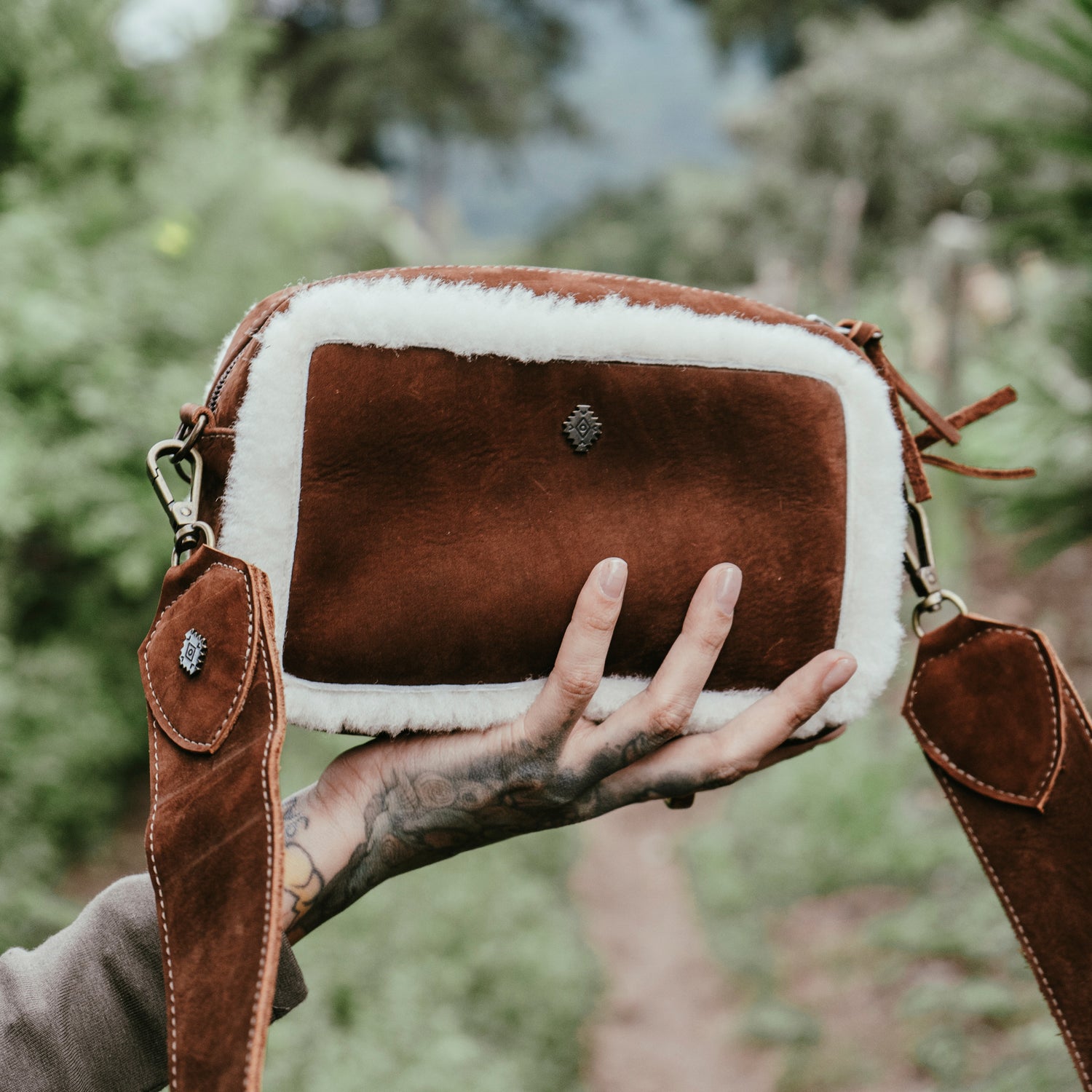In this image, a hand adorned with a tattoo on its top side holds a square-shaped purse outdoors. The hand, emerging from a gray sleeve on the bottom left of the image, presents three fingers gripping the purse with the other two fingers unseen. The purse features two brown straps, one on each side, connected by a gray hook. The purse itself is predominantly brown with white outer edging and a silver emblem in the center. The background highlights a green and gray, nature-based scenery, which appears blurred, drawing attention to the detailed foreground elements.